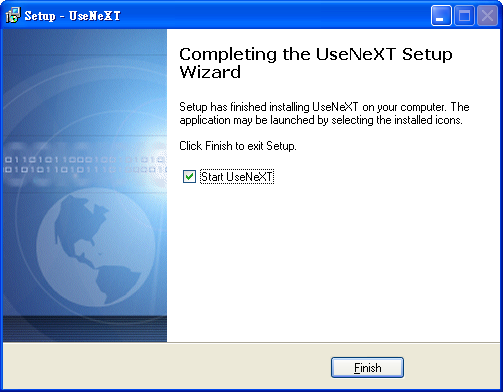This image features a single prominent object: a screenshot of a Windows computer installation dialog box for a program called "Use NEXT." The dialog box is centrally positioned and occupies the entire image. The box is designed with a blue and white color scheme, with additional light blue, green, tan, and a blue panel on the right that features an image of the Earth.

The dialog box displays the completion message: “Completing the Use NEXT setup wizard. Setup has finished installing Use NEXT on your computer. The application may be launched by selecting the installed icons. Click Finish to exit setup.” A notable green checkmark next to the text "Start Use NEXT" indicates that the application is ready to be launched once the setup is finished. The lower section of the box, in a cream color, contains the "Finish" button, marked for closing the setup wizard and starting the application. The upper panel of the dialog box includes typical window controls such as minimize, maximize, and close options in the top right corner.